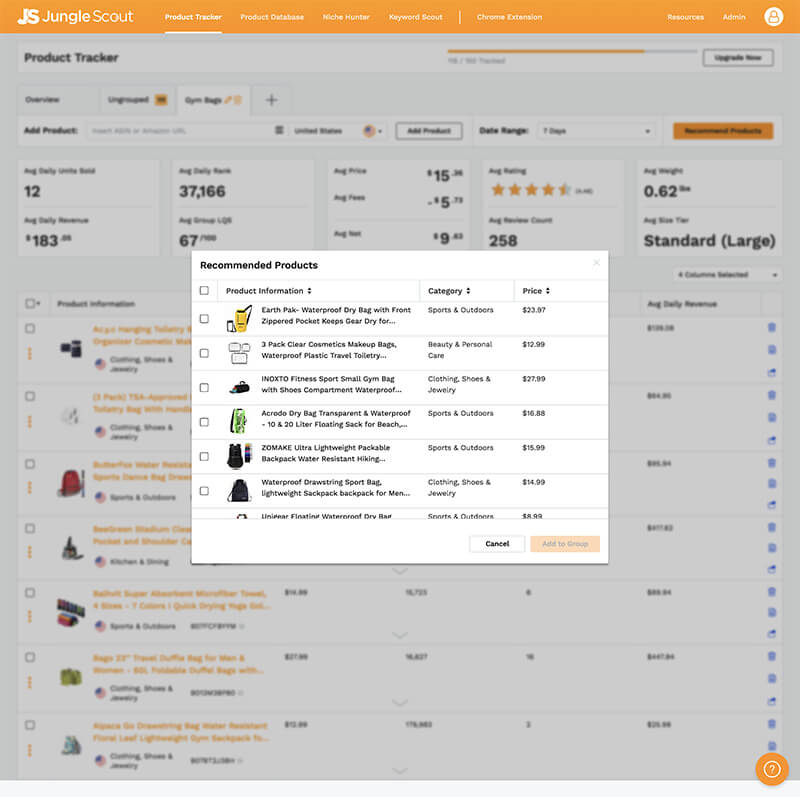The image showcases an advertisement sheet for Jungle Scout, featuring a prominent orange bar at the top. A pop-up window labeled "Product Tracker" is present, albeit slightly blurry, displaying a list of recommended products. The recommendations include detailed product information such as category and price. The text in the pop-up is colored in orange. Behind the pop-up, star ratings (ranging between 4 and 5 stars) are partially visible. The prices listed in the pop-up include $183, $67, $37, and $166. Different tabs are also noticeable, likely indicating various product sizes such as standard and large.